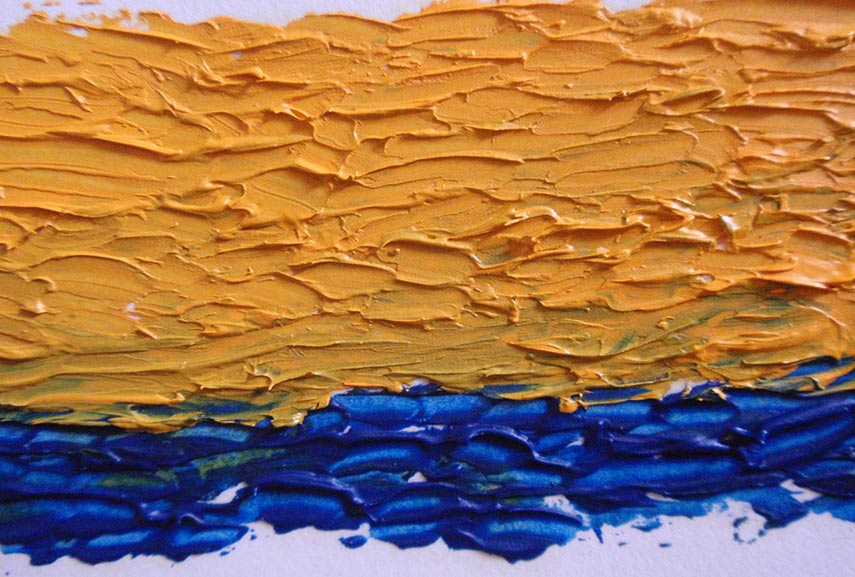This image is a close-up view of an abstract painting, likely created using thick, textured brush strokes or finger painting techniques. The composition features a primarily orange-painted surface covering the majority of the canvas, extending from the top down to roughly 80% of the image. At the bottom, there's a prominent strip of blue paint that adds contrast to the composition. The painting is characterized by substantial crevices, grooves, and texture, indicative of the heavy application of paint. Small unpainted areas of the canvas are visible at the top left and top center, revealing a light gray or white background. The edges of the image, both at the very top and bottom, show only a narrow strip of this unpainted canvas. The overall effect suggests a spontaneous, possibly childlike application of paint, with dynamic, short, and ridged strokes contributing to the artwork's chunky, tactile quality.